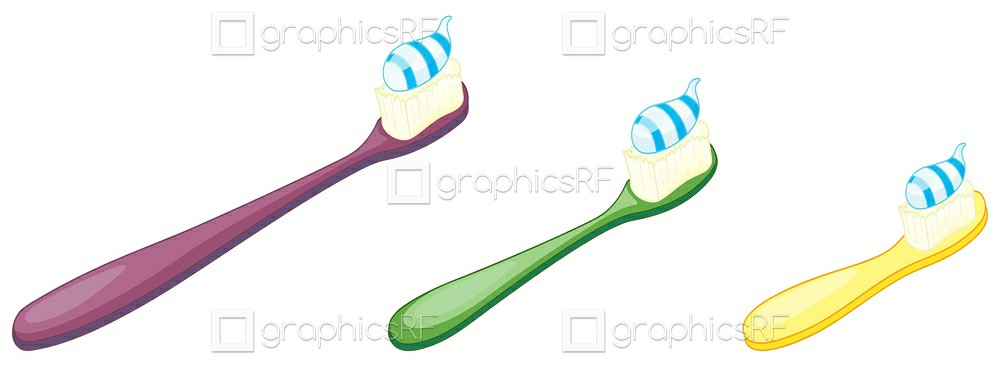This highly stylized, color illustration features three toothbrushes of varying sizes in a row, suggesting a nuclear family arrangement with the largest purple toothbrush on the left, a medium-sized green one in the middle, and the smallest yellow one on the right. Each toothbrush is angled diagonally, with the handles pointing toward the bottom left and the bristled heads toward the top right. Blue and white neatly striped toothpaste is artfully placed on the off-white bristles of each brush. The illustration is overlaid with multiple watermarks that read "Graphics RF," accompanied by a small empty checkbox, scattered in five different positions across the image. The background is a crisp white, emphasizing the vivid colors and clean design of the toothbrushes.